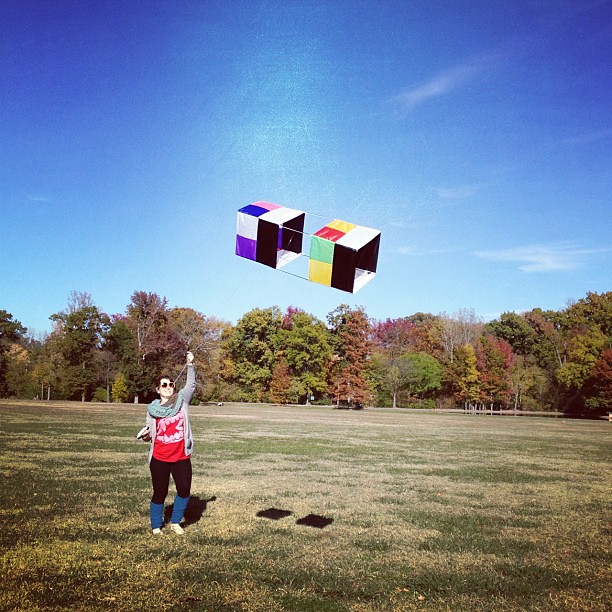In this vivid outdoor image, a woman stands in a grassy field that stretches across the bottom third of the picture. She is positioned towards the left side in the foreground, casting a soft shadow on the grass. The middle of the photograph is adorned with rows of trees displaying a beautiful array of fall colors, including red, yellow, and varying shades of green, with some trees having shed all their leaves. Above, the upper third of the image captures a bright blue sky dotted with wisps of clouds, and the sunlight enhances the lively atmosphere.

The woman, dressed warmly against the crisp autumn air, wears a gray open sweater over a red t-shirt featuring a white graphic design. A green scarf is wrapped around her neck, and she sports black leggings paired with blue leg warmers or knee-high socks, along with white sneakers. Short-haired and wearing dark sunglasses, she grips a kite string in her raised left hand. The kite, floating high in the sky, is a vibrant, rectangular prism. It features a myriad of colors on its panels, including pink, blue, white, purple, black, yellow, red, and green, with central sections made of clear material, allowing the blue sky to show through. The scene is a delightful capture of a serene moment of kite-flying under a sunny, fall sky.